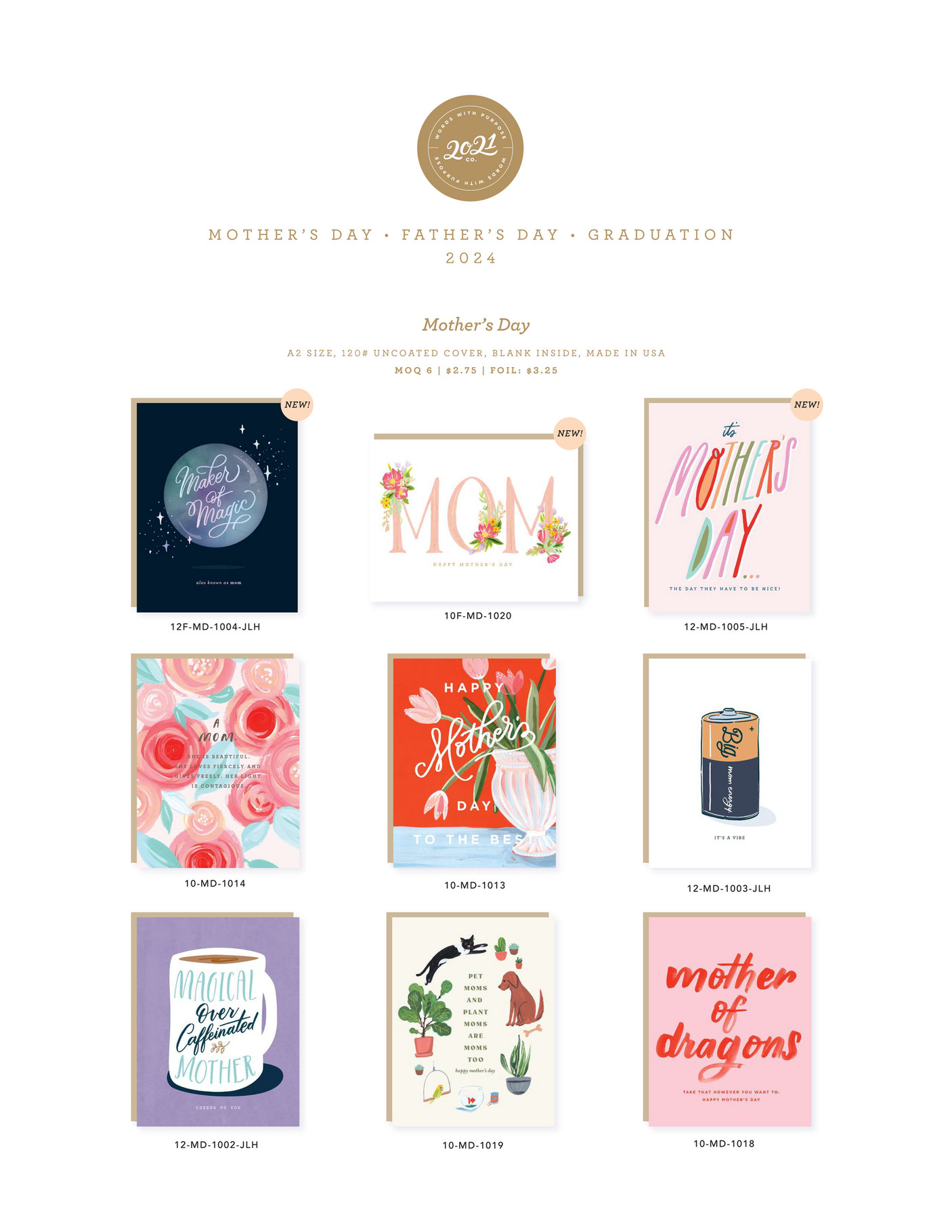The image depicts a poorly-resolutioned section atop of a display of greeting cards, featuring a circular brown emblem with an unintelligible white cursive inscription which could possibly be "L-O-L-1." Below this emblem, white text on the brown background reads: "Mother's Day, Father's Day, Graduation, 2024, Mother's Day."

Further details are listed below in smaller text: "A2, Size 120, #Uncoded, Cover, Blank Inside, Made in USA, MOQ-6, 275 Foil, 325."

The main section showcases an array of nine Mother's Day cards organized into three rows of three cards each. The cards in the first row read: "Maker of Magic," "Mom," and "It's Mother's Day, the day they wave to the [illegible text]." The cards in the second row read: "A Mom [with additional small print text]," "A Happy Mother's Day to the Best," and "Big Mom Energy" featuring a battery illustration.